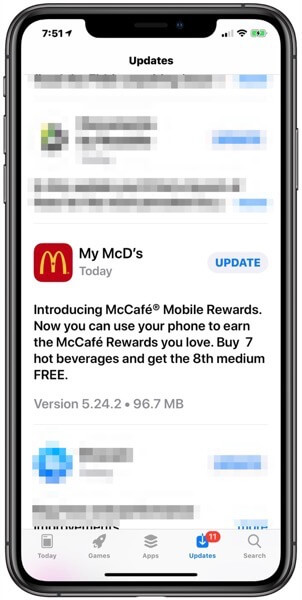A close-up image of a smartphone displaying an app update notification for McCafe mobile rewards. The phone has plastic edges with a 7.31mm top bezel. The screen shows full Wi-Fi connectivity and a fully charged battery icon. The app notification is slightly pixelated and difficult to read, saying "Introducing McCafe mobile rewards, now you can use your phone to earn the McCafe rewards you love. Buy 7 hot beverages and get the 8th medium free." The version 5.2.42 update is 96.7 megabytes in size. Icons for games, apps, and updates can be seen on the left side of the screen, along with a blue square with the number 11. There's also a magnifying glass icon indicating a search function at the bottom of the screen. The edges of the phone are described as very black or grey with some buttons visible on the sides. The overall image quality is quite blurry, making the text and some details hard to discern.